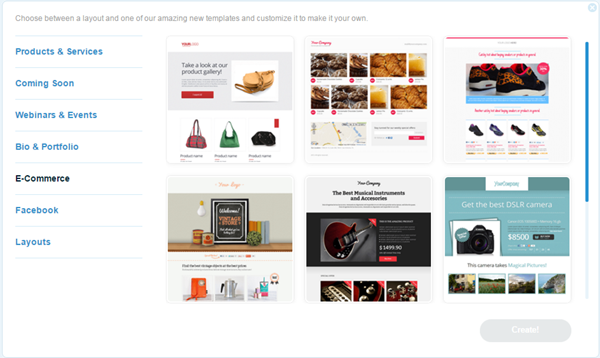This image is a screenshot of a website displayed in landscape mode, enclosed by a thin blue border. In the far upper right corner, there is a blue circle with a white 'X' inside. Moving to the top left, there is a message in light gray font that reads, "Choose between a layout and one of our amazing new templates and customize to make it your own."

Below this header, a vertical column runs along the right side of the screen, segmented into various sections, each with thin blue borders on the top and bottom. The sections are labeled as follows: Product and Services, Coming Soon, Webinars and Events, Bio and Portfolio, and E-commerce, with the E-commerce section being highlighted in black while the others remain blue. Further down, the labels Facebook and Layout can be seen.

The main body of the website, positioned slightly to the right, features two rows of three small squares, presumably template previews. The top row includes images of various products: purses on the left, an indistinct image with a partial map in the center, and shoes on the right. The bottom row features additional product images: an unidentifiable object on a shelf to the left, a guitar and related images in the center, and an image related to a camera on the right, complete with descriptions and tests.

In the lower-right corner, the image has a light gray button with white text that is difficult to discern.